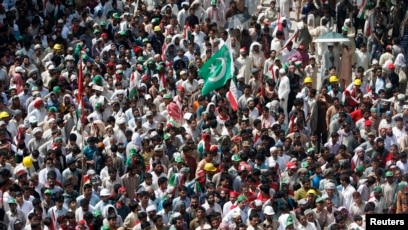This overhead photo captures a densely packed crowd of people, predominantly of Middle Eastern or Indian descent, judging by their skin tones and attire. The image conveys a sense of either a significant protest or a bustling demonstration. A key feature in the center of the crowd is a large green flag bearing a white crescent moon and star, hinting at its probable Muslim affiliation. There is also a secondary flag displaying red, white, and possibly black stripes, partially obscured by the image's blur. Scattered throughout the multitude are individuals wearing yellow hats; specifically, nine are counted. Additionally, several people sport green hats. The bottom right corner of the photograph features a black bar with the word "Reuters," suggesting the image's newsworthy nature and likely use in a Reuters article. The sheer number of participants makes the ground beneath them invisible, emphasizing the magnitude of the gathering.